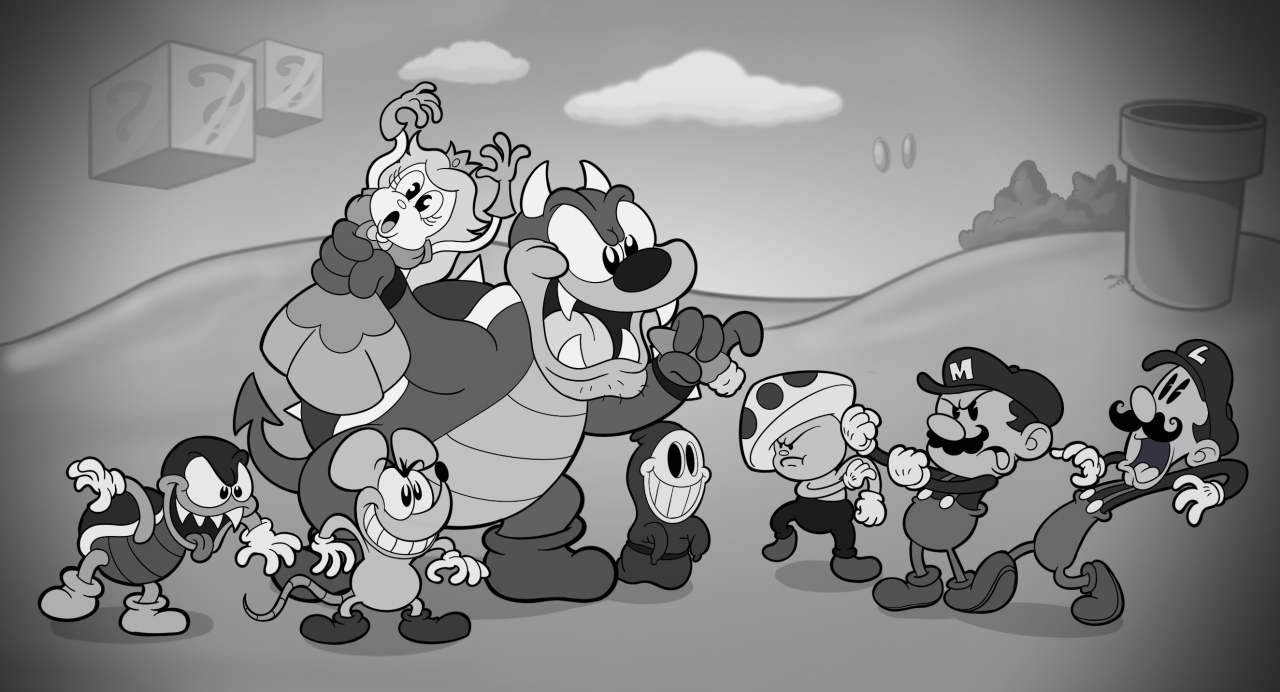This detailed black-and-white image depicts characters from the Mario franchise in a 1920s cartoon style reminiscent of "Steamboat Willie." The scene unfolds on rolling grass hills with floating question mark blocks and cylindrical coins in the air, and fluffy white clouds in the sky. There is also a pipe on one of the hills near Luigi.

On the right, Mario stands with his fists up, ready to fight. He wears grey suspenders, dark grey shoes, a black undershirt, a black 'M' cap, and white gloves. Next to him, Luigi looks horrified with his mouth open, revealing his tongue. He's dressed similarly, with grey suspenders, large grey shoes, a black 'L' cap, and white gloves. Toad, slightly to the left, rubs his right arm as he prepares for the confrontation. He sports a mushroom cap with black spots, black trousers, and smaller dark grey shoes.

Central to the scene is Bowser, a large, menacing turtle-like figure with a dark grey outline, white horns, black pupils, a black nose, four white fangs, and a stubbly chin. He laughs menacingly while holding a cigarette. His body has a lizard-like texture with lines along the underside. In his left hand, he clutches Princess Peach, who is flailing her arms in distress. Peach has short grey hair, a small crown, black pupils, and a grey dress.

Surrounding Bowser are other iconic adversaries. To his left is a Shy Guy with black, hollow eyes, a wide mouth, and a dark grey cape secured with a black belt. Next to the Shy Guy is a mouse-like creature with a black nose, black pupils, white gloves, black shoes, and a menacing smile, featuring a long tail. Further to the left is a Goomba, a small turtle-like enemy with mid-grey legs, black pupils, and a black shell with a white outline.

Together, the characters create a scene that blends nostalgia with the iconic imagery of the Mario universe, all amidst detailed and dramatic black-and-white artistry.